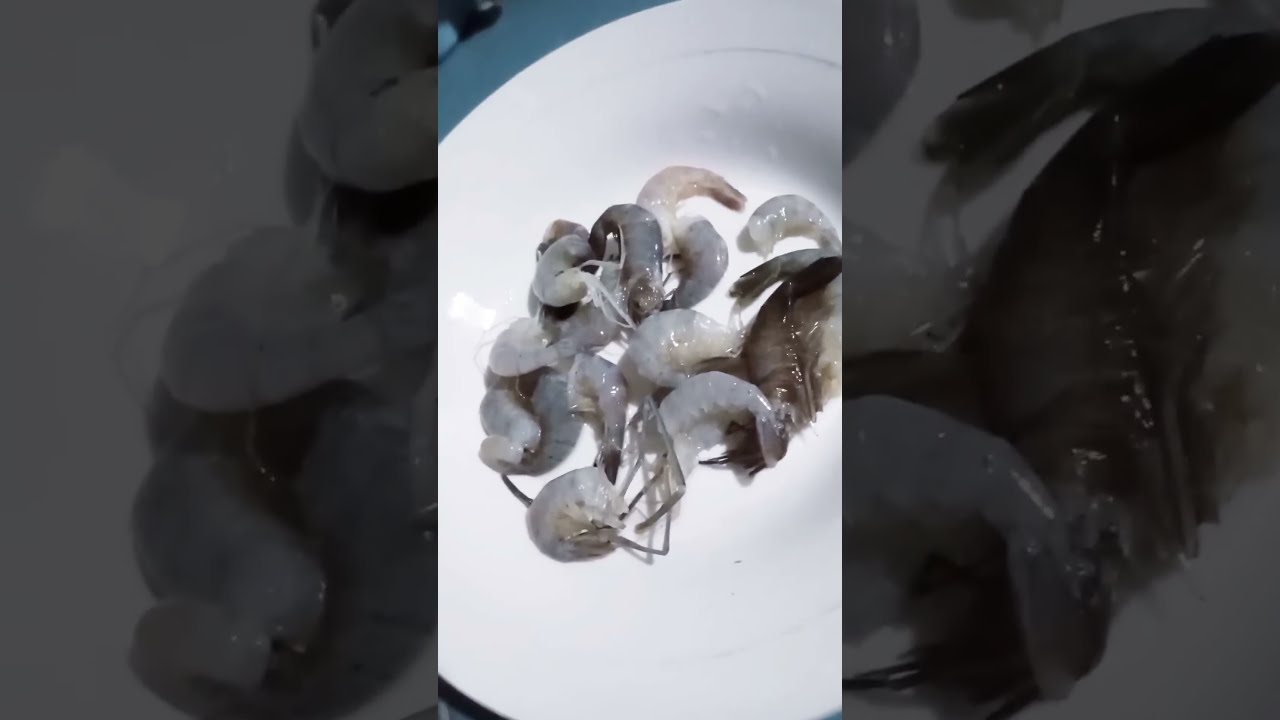This image captures a plate of raw shrimp, predominantly grey with some displaying shades of whitish-pink and dark grey. These shrimp, which still bear their legs, appear partially peeled and presented on a bright white plate with a silver rim that curves inward, resembling a pasta plate. Some of the shrimp are almost transparent, and they're arranged in such a way that they seem ready to slide off the plate, which is slightly tilted towards the lower left corner. The background in the upper left is a dark blue, though it’s unclear if this is part of the plate or the surface it rests on. Additionally, the image features enlarged, tinted close-ups on the left and right sides, which offer a detailed view of the shrimps' texture and color, enhancing the central image's composition.